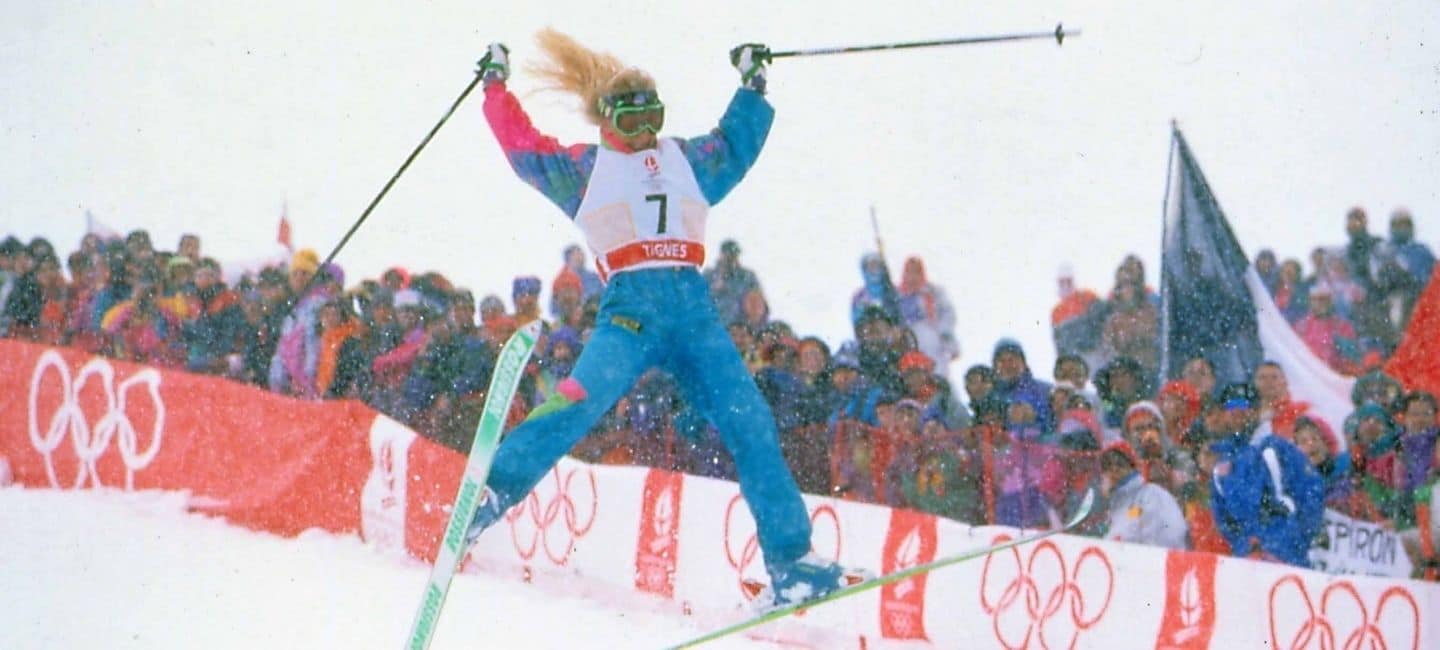This photograph, taken at a Winter Olympic skiing event from the 1980s or 90s, captures a skier in midair with her poles raised triumphantly. She wears a retro blue, green, and pink snowsuit along with green goggles, complementing her blonde hair. The skier, identified by the number 7 on her bib, seems to be either jumping or celebrating, with her skis off the snow. The backdrop is a snowy, almost whiteout scene, adding to the wintry atmosphere. Spectators, clad in heavy winter jackets, goggles, and beanies, line the course behind an orange banner featuring the Olympic rings, with "Tignes" clearly visible on it. Among the crowd, some hold flags, including a noticeable French flag, and many have signs showing their enthusiasm and support for the event. The overall vibe reflects a vibrant and spirited Olympic moment characterized by the skier's dynamic pose and the engaging crowd.